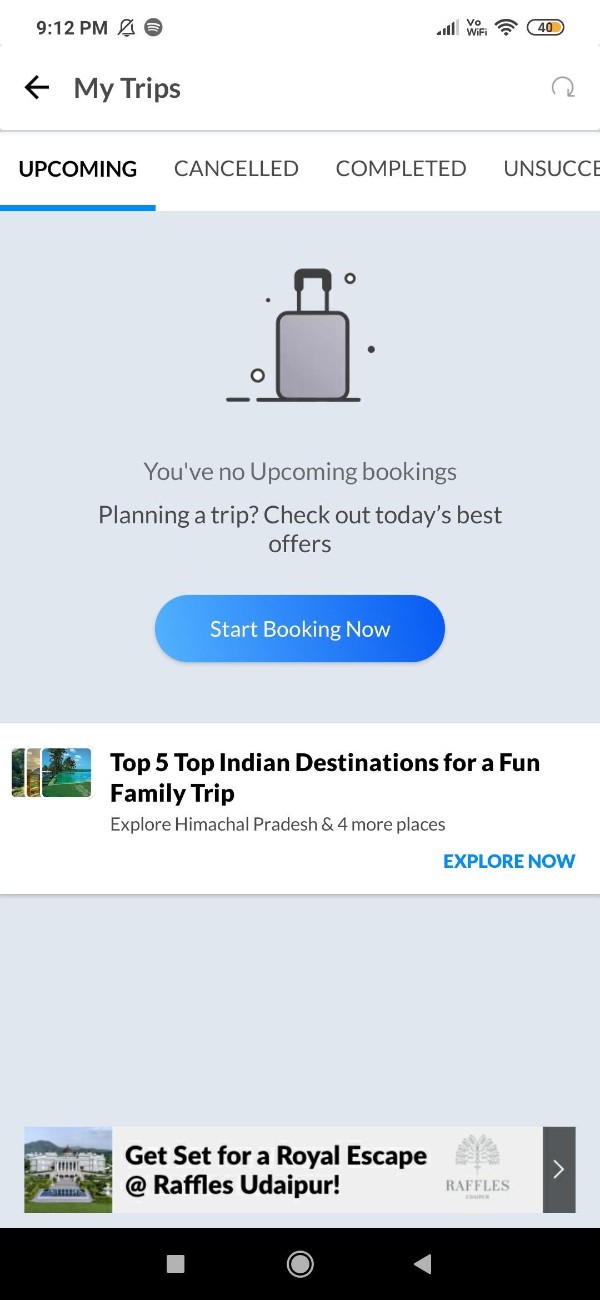**Detailed Caption:**

The screenshot depicts a mobile phone interface with a white background and black text. At the top left corner, it displays the time "9:12 p.m." followed by a bell icon with a slash through it, indicating notifications are muted. Next to that is an icon likely representing Spotify, which shows a gray circle with a black interior. The right side of the top bar features full Wi-Fi coverage bars and a battery icon inside a black circle with the number "40" and a small orange segment, suggesting the battery is at 40%.

Below the top bar, there's a navigation arrow pointing left with the label "My Trips" next to it and a three-quarter gray circle on the right. Underneath this, the interface shows several tabs: "Upcoming" highlighted in black and underlined in blue, with "Cancelled", "Completed", and "Unsuccessful" in lighter black text.

The main content area has a gray squared background featuring a suitcase icon outlined in black with gray interior bubbles around it. The text inside the square reads, "You have no upcoming bookings." Beneath, it suggests, "Planning a trip? Check out today’s best offers," accompanied by a clickable blue button with "Start Booking" in white text.

Further down, there's a section with an image captioned in dark black text, "Top 5 Indian Destinations for a Fun Family Trip," followed by gray text that reads, "Explore Himachal Pradesh and 4 more places." A blue "Explore" link appears to the right of this description.

At the bottom of the screen, the text reads, "Get set for a royal escape," followed by a black bar containing gray icons of a square, a circle, and a triangle pointing left.